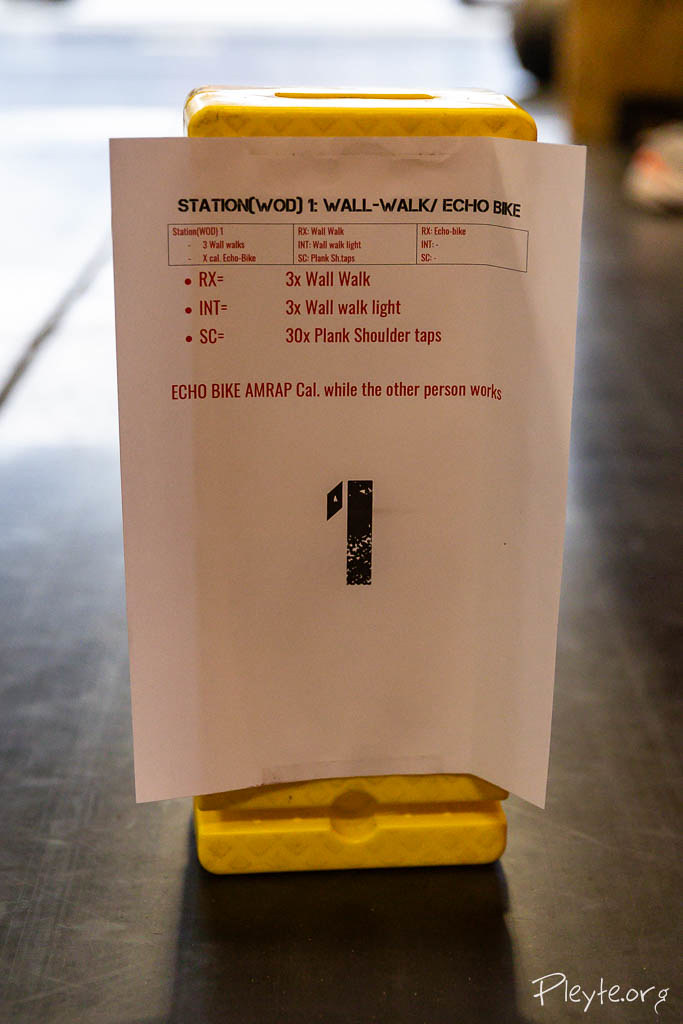The image showcases a close-up of a piece of white printer paper taped to a yellow plastic block, which is placed on a wooden table. The paper is titled "Station W.O.D. 1 Wall-Walk-Echo-Bike" in both black and red lettering. Below the title, there are three bullet points with associated codes: "Rx equals 3x Wall-Walk," "Int equals 3x Wall-Walk Light," and "Sc equals 30x Plank Shoulder Taps," all in red text. Under these instructions, it reads "Echo-Bike AMRAP (as many reps as possible) Cal while the other person works" in black. A large number "1" is printed at the bottom of the page. The image also has a faint watermark on the bottom right corner, stating "P-L-E-Y-T-E.org."